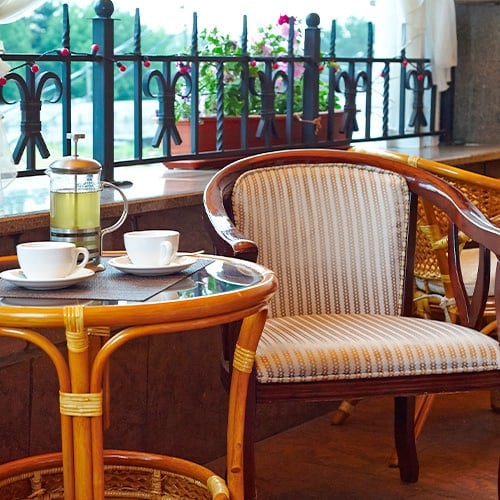This photorealistic image depicts a charming cafe setting, likely on a patio. The focal point is a small table made of brown wicker with a glass top. On the table, two white mugs rest on saucers alongside a French press filled with green tea. Dominating the seating area is a wooden armchair with arms and a cushion featuring satiny, striped beige upholstery. Another chair is partially visible behind it.

The scene is framed by a low stone wall topped with a decorative black iron fence, adorned with a potted plant that has small, delicate pink flowers cascading around the ironwork. The background includes a large plate glass window, possibly looking out over a yard, adding to the cozy ambiance of the cafe.